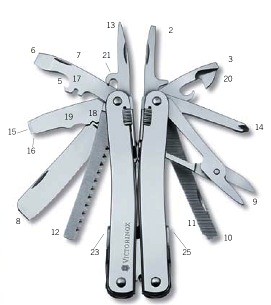This image depicts a detailed close-up of a multifunctional pocket tool, resembling a Swiss Army knife or Leatherman, with 25 different stainless steel attachments. The tool, which appears silver and is brand-named Victorinox, showcases a variety of blades and utilities including scissors, a bottle opener, a can opener, various types of knives, a file, a saw, and both flathead and Phillips head screwdrivers. The attachments are neatly spread out in a circular fashion against a white background, allowing each tool to be visible. Each tool is marked with numbers ranging from 2 to 25, with lines pointing to the corresponding attachments, creating a diagram-like presentation. The knife handle is inscribed with "Victorinox" in vertically ascending letters, and the tools are connected by small metal rivets ensuring they remain secured.